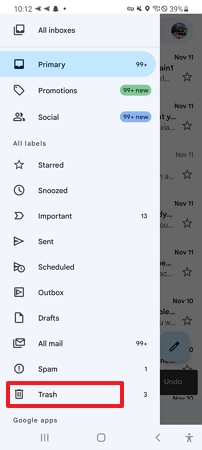This screen capture displays a cell phone using the Gmail app, specifically focusing on the side panel menu. The phone's status icons in the top right-hand corner indicate a 39% battery level, a circle with a line through it (possibly indicating do not disturb mode), a Wi-Fi signal, a geolocation symbol, a muted microphone, and a Bluetooth symbol.

In the upper left corner of the screen, the time reads 10:12 AM. Adjacent to the time are two left-pointing arrows followed by a Snapchat icon and a small dot.

Beneath these, the image shows the expanded side panel of the Gmail app in detail. The panel lists various folders and labels with corresponding symbols:

- **All Inboxes**: Represented by a mailbox folder icon.
- **Primary**: Denoted by a singular mailbox folder icon with "99+" indicating unread emails.
- **Promotions**: Marked by a tag symbol and also showing "99+" unread emails.
- **Social**: Indicated by a two-people symbol and listing "99+" unread emails.
- **All Labels**: Simply titled without a symbol.

Following this are several secondary labels and their icons:
- **Starred**: Marked by a star symbol.
- **Snooze**: Displayed with a clock symbol.
- **Important**: Denoted by an arrow icon and indicating 13 unread emails.
- **Sent**: Represented by a paper plane icon.
- **Scheduled**: Shown with a paper plane and a timer.
- **Outbox**: Indicated by a play button icon.
- **Drafts**: Represented by a paper with a folded corner icon.
- **All Mail**: Depicted with multiple pieces of mail and showing "99+" unread emails.
- **Spam**: Marked by a stop sign with an exclamation point, indicating 1 spam email.
- **Trash**: Highlighted in red and depicted by a trash can symbol, showing 3 items in the trash.

This detailed breakdown captures the various elements and status indicators present in the Gmail sidebar, providing a comprehensive view of email organization and phone status.